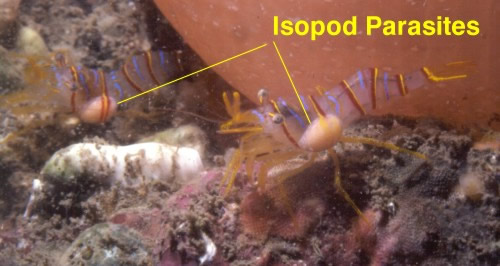In this color underwater photograph, two translucent crustaceans are depicted crawling on a sandy sea floor. Resembling crayfish but lacking claws, these creatures have elongated, worm-shaped bodies with distinctive thin yellow, brown, and red stripes along their backs. They possess yellow legs and prominent snouts or noses, with two noticeable black eyes on their heads. Within the transparent sections of their bodies, beige bubble-like structures are evident, likely the focus of the bold yellow text that reads "isopod parasites." This text, located in the upper right corner, is accompanied by yellow arrows pointing to these bubbles, suggesting they are parasitic organisms inside the crustaceans. The background features a large, indistinct red circular object, adding a contrasting element to the scene.